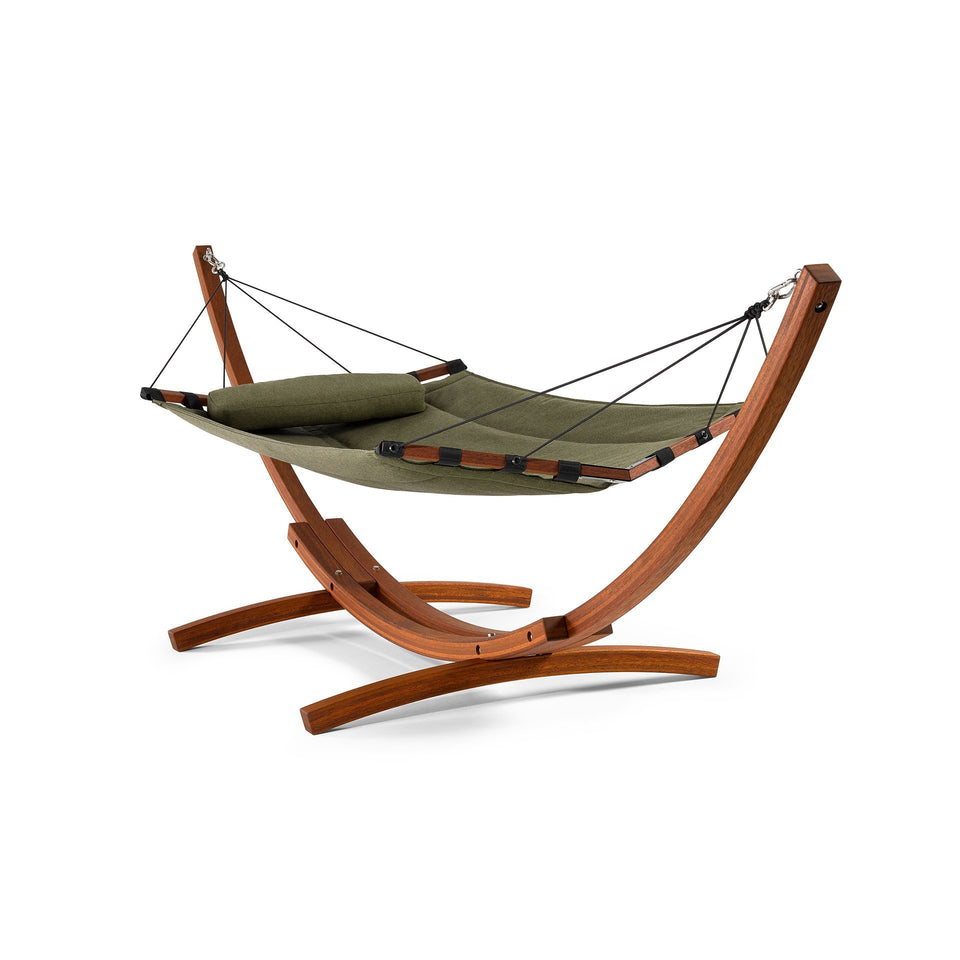This image showcases a beautifully constructed small hammock designed for comfort and elegance. The hammock bed is a rich green color, made of weatherproof quilted canvas, and includes a matching mini pillow for head support. It is suspended by black nylon ropes connected to four strings on each side, securing it to handcrafted wooden pieces that keep it spread out. The entire hammock is supported by a unique U-shaped wooden frame, made from four carefully joined sections to form a large, banana-shaped arch. Two smaller U-shaped wooden supports provide a stable base. The background is a plain, solid white, emphasizing the meticulous craftsmanship and inviting comfort of the hammock. The frame is fastened together with numerous screws, adding to its sturdy construction, ensuring that it’s both aesthetically pleasing and functional.